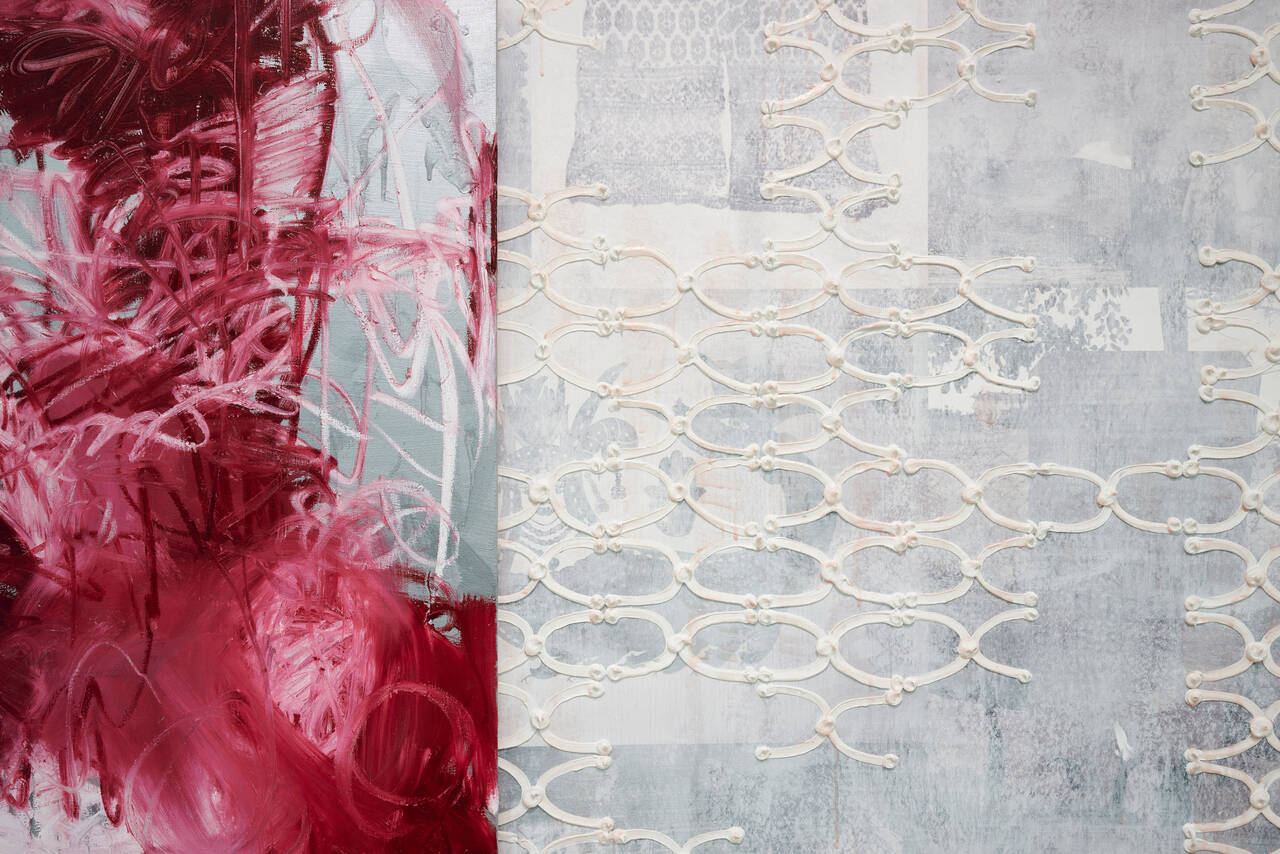The horizontal image resembles an abstract painting or artistic design. Dominating the left side is a vibrant and chaotic mixture of red and pink paint, appearing randomly scratched on and smeared around, creating a blur of colors that almost blend into a lighter, pinkish hue. The light blue background is mostly obscured by this mass of paint. On the right side, the background transitions to a light gray-beige hue, hosting a series of squarish and oval-shaped white patterns. These white ring-like shapes interlink in some places and remain open in others, resembling chain links or possibly the remains of tiles that have been ripped off a wall. The whole composition is visually intriguing, with its stark contrast between the chaotic left and the more structured, patterned right. There is no text, maintaining the focus on the enigmatic artistry.